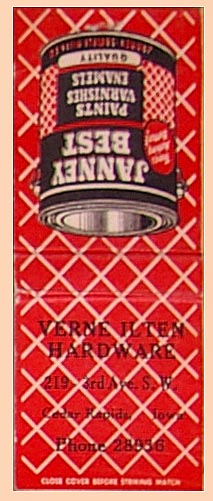The image depicts a vintage matchbook advertisement, predominantly red with a crisscross pattern of white stripes. The matchbook appears to be partially open, revealing two sides: one oriented normally and the other upside down as if designed to fold into an A-frame stand. The right-side-up section displays the text "Vern Ilton Hardware, 219 3rd Avenue SW, Cedar Rapids, Iowa," with an old-fashioned phone number "28938." The upside-down section features an image of a paint can labeled "Janney Best Paints, Varnishes, and Enamels." The bottom of the matchbook hints at its age with the instruction, "Close cover before striking." This artifact, likely from the early 20th century, presents a quaint snapshot of past marketing strategies and product design.